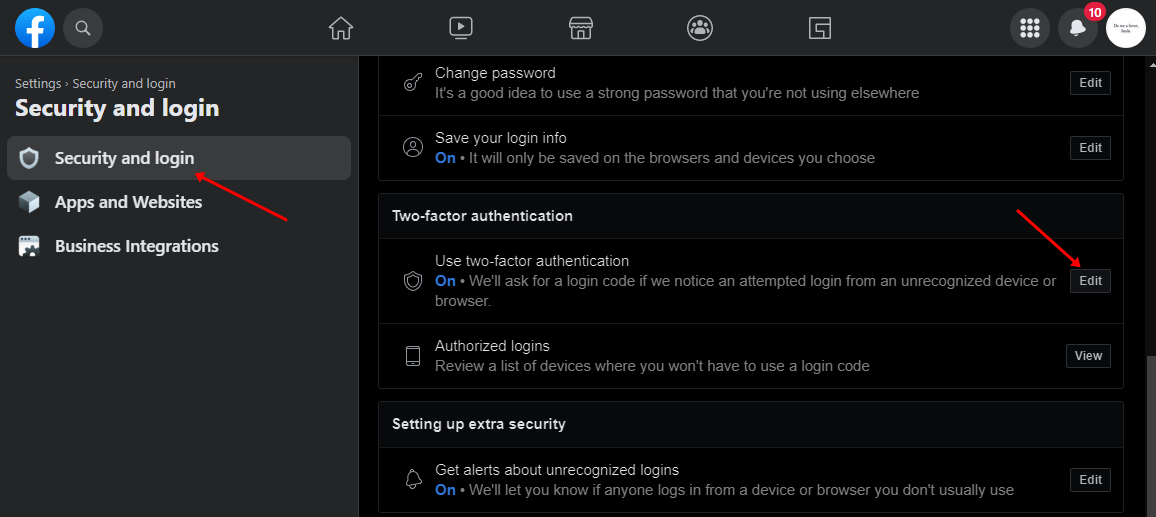The image captures a screenshot of the Facebook settings page with a focus on security and login features. In the top left corner, the recognizable blue circle with a white "F" signifies the Facebook logo. Adjacent to it, a red button and another button are positioned on the top right side of the image. The top menu includes navigation options: Home, Videos, Marketplace, Groups, Reels, and Menu. Additionally, there is a Notification icon displaying a red circle with the number 10, indicating 10 new notifications, and a white profile icon.

On the left side, a side menu lists various options: Security, Settings, Security & Login, Security & Login, Security & Login, Apps & Website, and Business & Integration. A prominent red arrow points specifically to Security & Login.

The main section of the page has a black background with white text, except for instances where "ON" is highlighted in blue. At the top, the title "Change Password" is displayed, along with the advice: "It's a good idea to use a strong password that you are not using elsewhere." Below this, there is a feature titled "Save Your Login Info," which is turned "ON" and explained as being saved only on selected browsers and devices.

Further down, "Two-Factor Authentication" is introduced with an explanation that it is enabled ("ON") to request a login code for any attempts from unrecognized devices or browsers. A red arrow points to the "Edit" button for this feature.

Additional settings include "Authorized Login" with a "View" button that allows users to review devices where a login code isn't needed, and "Setting Up Extra Security," where "Get Alerts" is enabled ("ON") to notify the user if someone logs in from an unfamiliar device or browser.